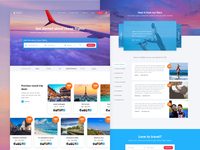This is a blurry screenshot likely taken from a laptop, desktop, or tablet. The screenshot appears to be from a travel or booking website, featuring a collage of images and text. The main cover image showcases a breathtaking view from an airplane window, capturing the wing of the plane as it soars above the clouds during either sunrise or sunset. The sky is adorned with a stunning gradient of purplish hues transitioning into the golden yellows typical of a setting sun. Below this main image are smaller, indistinct visuals, including a recognizable silhouette of the Eiffel Tower and other exotic landmarks. On the right side, there are additional images and accompanying text, possibly blog posts or travel adventure descriptions, although the text is too blurred to read clearly.